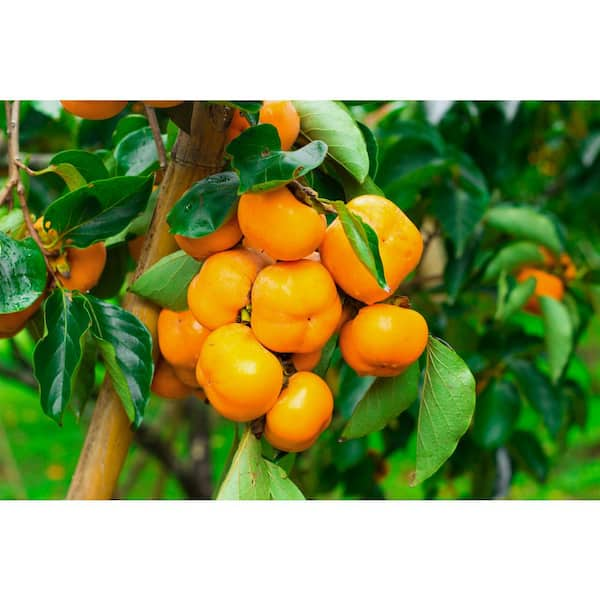The photograph captures a vibrant persimmon orchard. At the center of the image, amidst a backdrop of verdant foliage, is a cluster of ripe, orange persimmon fruits that resemble rounded tomatoes growing in bunches. These persimmons, with their cube-like shapes, hang from a tree with a robust brown stem. The tree is adorned with long, pointy dark green leaves that have a smooth texture, adding a lush contrast to the vivid fruit. To the right, another tree with persimmon fruit appears blurred, enhancing the focus on the central cluster. The bottom of the photo reveals a patch of green grass, grounding the image in the natural setting of an orchard.